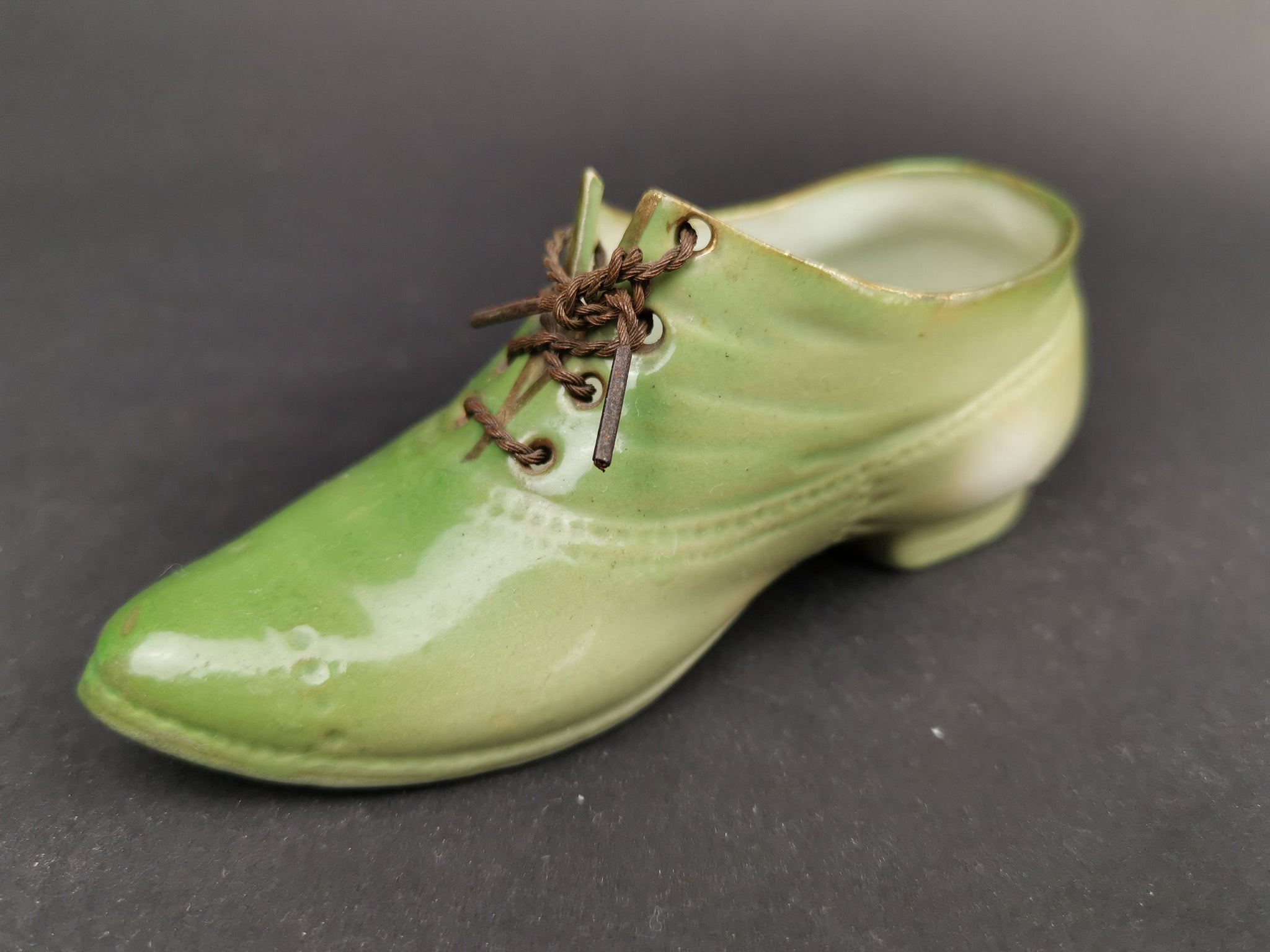This image features a detailed rendering of an old-fashioned woman's shoe crafted from porcelain or ceramic. The shoe, prominently centered against a black background, showcases various shades of pale celery green, which intensify at the toe and fade towards the heel. Highlighting its decorative purpose, the shoe is adorned with a brown, vintage leather shoelace that appears worn, adding an authentic, antique feel. Subtle detailing mimics stitching along the sides and front, enhancing the shoe's realistic impression. The interior of the shoe is a creamy white, with a touch of brown along the edges, and the presence of a tiny heel at the back completes its classic design. The overall shiny finish of the porcelain gives it a polished look, making it a visually captivating piece.